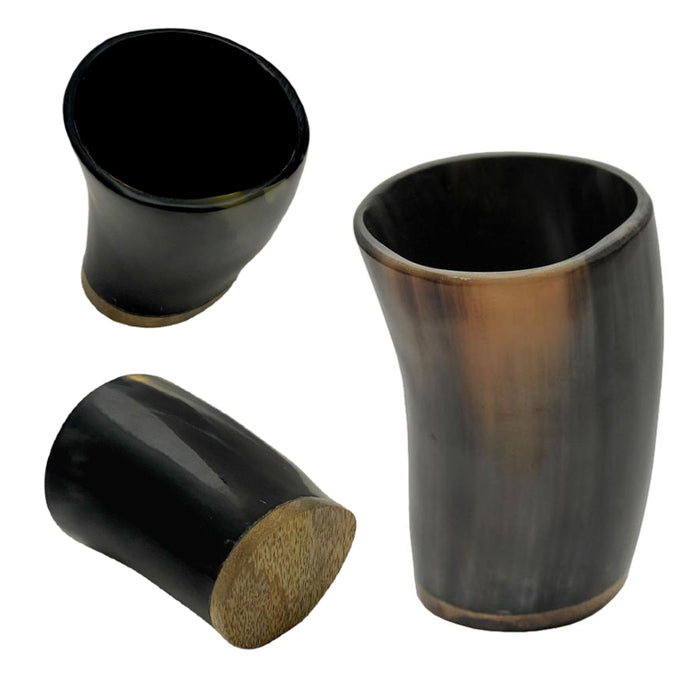This image features three modern-looking canisters with a white background in the top right corner. The largest canister is positioned on the right side of the image, standing upright, and it showcases a dark gray exterior with a light brown trim around the bottom. The interior of this canister appears pitch black. The second canister, located at the top left, is slightly tilted towards the camera. It has a similar dark gray outer surface and a light brown bottom trim; its top part reveals a completely black interior as well. The smallest canister is at the bottom left, lying on its side. It has a dark gray, almost black exterior and a wooden, light brown bottom, displaying a subtle grain texture. Each canister appears to be made of or aesthetically similar to smoothed-out wood with a glossy finish, adding a touch of shine. There are also suggestions that the canisters might be artistic renditions, as indicated by some irregularities in shape.